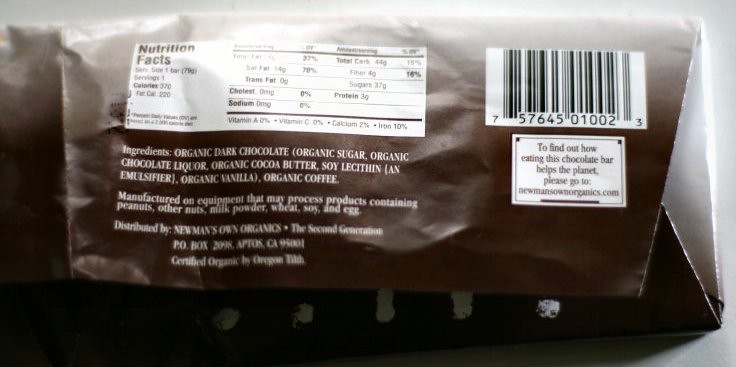The image is a detailed close-up of the back of a Newman's Own Organics dark chocolate bar package. Prominently displayed on the left side is a nutrition facts label. Adjacent to the label, on a dark background, is an ingredient list in white text, stating: "Ingredients: Organic dark chocolate (organic sugar, organic chocolate liquor, organic cocoa butter, soy lecithin [an emulsifier], organic vanilla, organic coffee)." Below the nutrition information is additional white text indicating the chocolate was manufactured on equipment that may process various allergens, and providing distribution information by Newman's Own.

On the right side of the package, there's a black and white striped barcode with the number "757645010023" beneath it. Directly below the barcode is a white label encouraging customers to visit "newmansownorganics.com" to learn how purchasing the chocolate helps the planet.